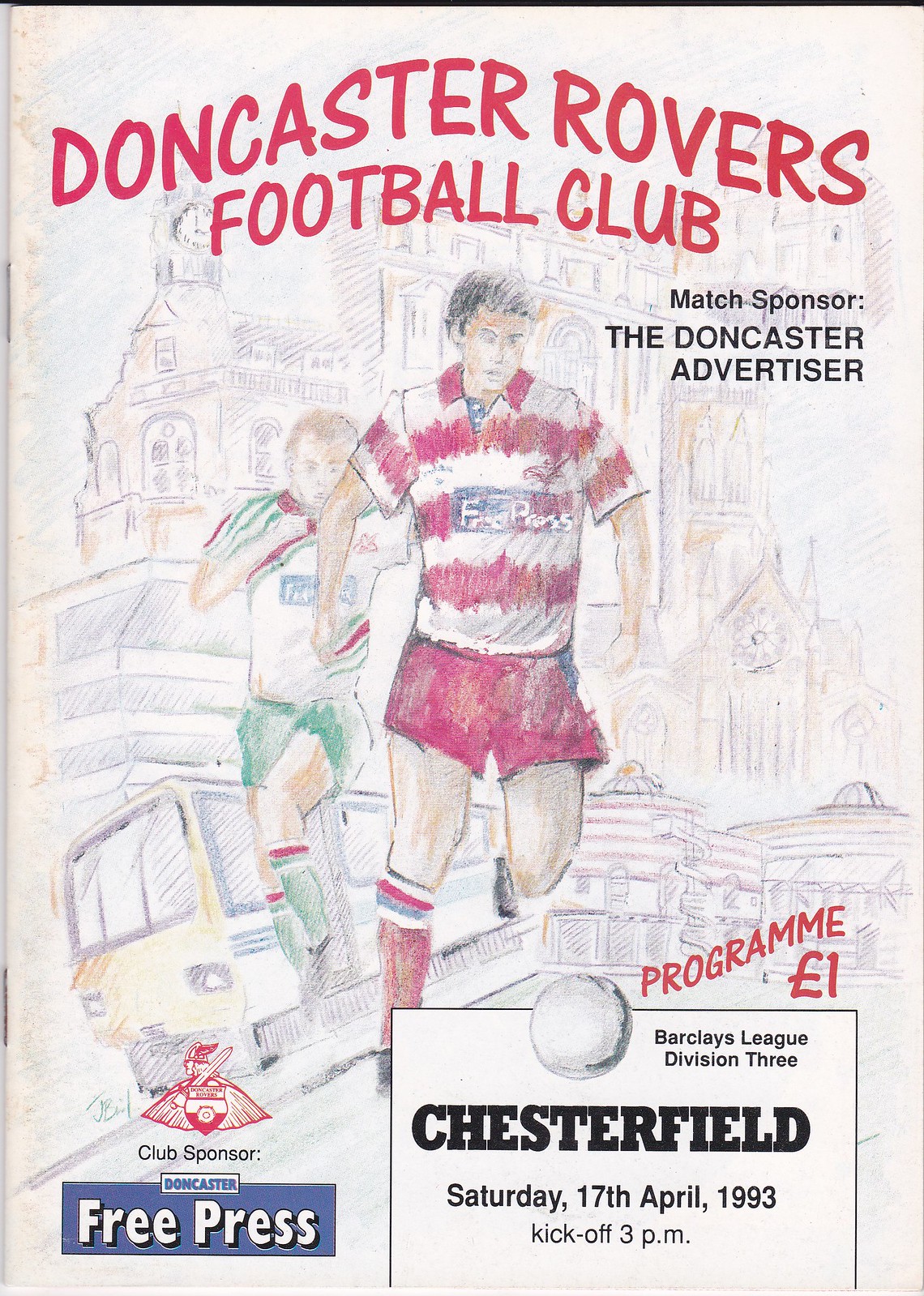The cover of the Doncaster Rovers Football Club's European Football Program from April 17, 1993, features a detailed sketch with an old-fashioned aesthetic reminiscent of early 1900s illustrations. At the top, in pinkish-red letters, it reads "Doncaster Rovers Football Club," with a smaller black-font note to the right indicating the match sponsor, Doncaster Advertiser. The main image depicts two footballers mid-action: one in a red and white striped shirt with red shorts, who is being pursued by another player in a white jersey with green stripes on the shoulders and green shorts. The scene is set against a backdrop of city elements, including a car, buildings, a train on rails, and a barely discernible older building with a clock. At the bottom, it specifies the upcoming match details: "Chesterfield, Saturday, 17th April, 1993, kickoff, 3 pm," and notes the club sponsor, Free Press, alongside the program's price listed as one lira.